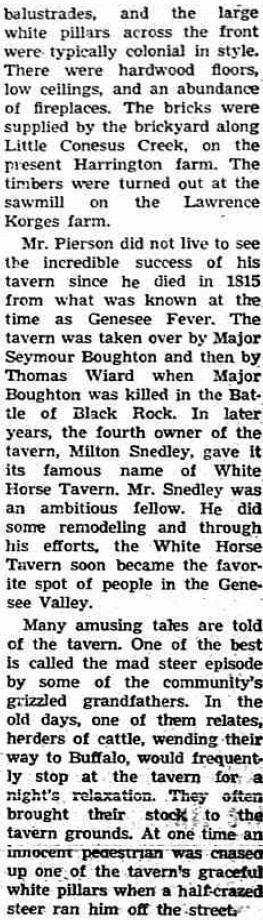This image is an excerpt from a print document with black text on a white background, featuring a detailed narration about an old tavern. The text describes a historical tavern known for its colonial architecture, characterized by large white pillars, balustrades, hardwood floors, low ceilings, and numerous fireplaces. The construction materials were locally sourced with bricks supplied by the brickyard along Little Canesis Creek and timbers from the sawmill on the Lawrence Corg's Farm. The original proprietor, Mr. Pearson, tragically did not witness the tavern's success as he passed away in 1815 from Genesee Fever. The tavern was later managed by Major Seymour Boughton, who perished in the Battle of Black Rock, followed by Thomas Weirard, and eventually Milton Sneedly. Sneedly, the fourth owner, remodeled the tavern and christened it the White Horse Tavern, establishing it as a beloved locale in the Genesee Valley. Among the many tales from this establishment’s vibrant history is the "Mad Steer episode," recounting a chaotic scene where a pedestrian was chased up one of the tavern's white pillars by a frenzied steer. This column is part of a larger narrative and includes three related photographs.